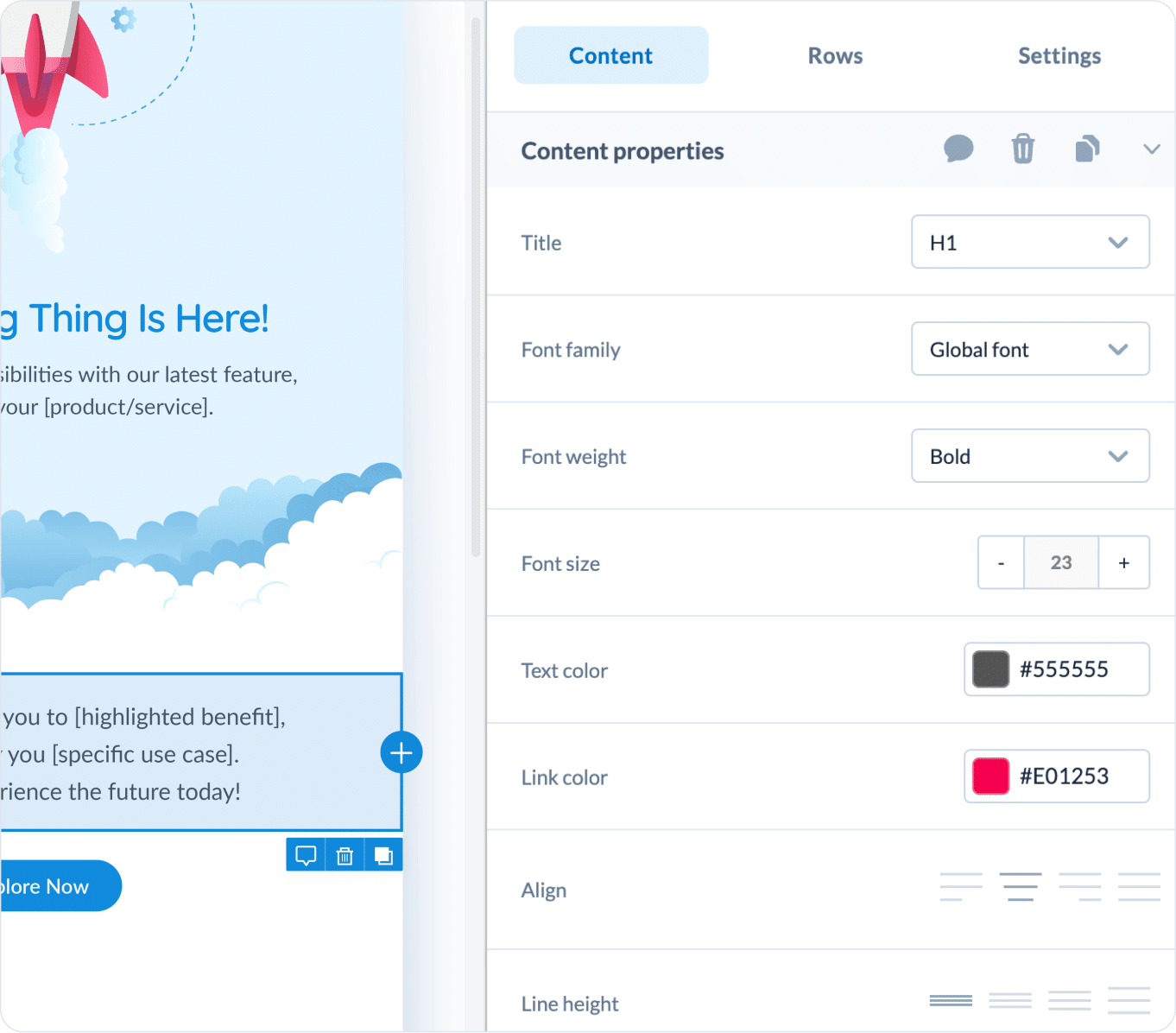The image features a partially cropped area on the left, displaying a portion of clouds and a serene, blue sky. Superimposed over this scenic backdrop are the words: "The future today," highlighting some of the latest features, products, services, and benefits.

On the right side of the image, the background is predominantly white. At the very top, there is a light blue box with selected content inside. To the right of the blue box, the word "rose" is visible, followed by "sentence" to its immediate right. Below this, the section labeled "Content Properties" is visible, containing various interactive elements: a text box, a trash can icon, and another unidentified icon.

Further down, under the "Title" section, there is an editable box with a drop-down menu set to "H1." Below that, the "Font Family" section features another drop-down menu displaying "Global Font." Finally, there is a "Font Weight" option, indicating additional customization settings.